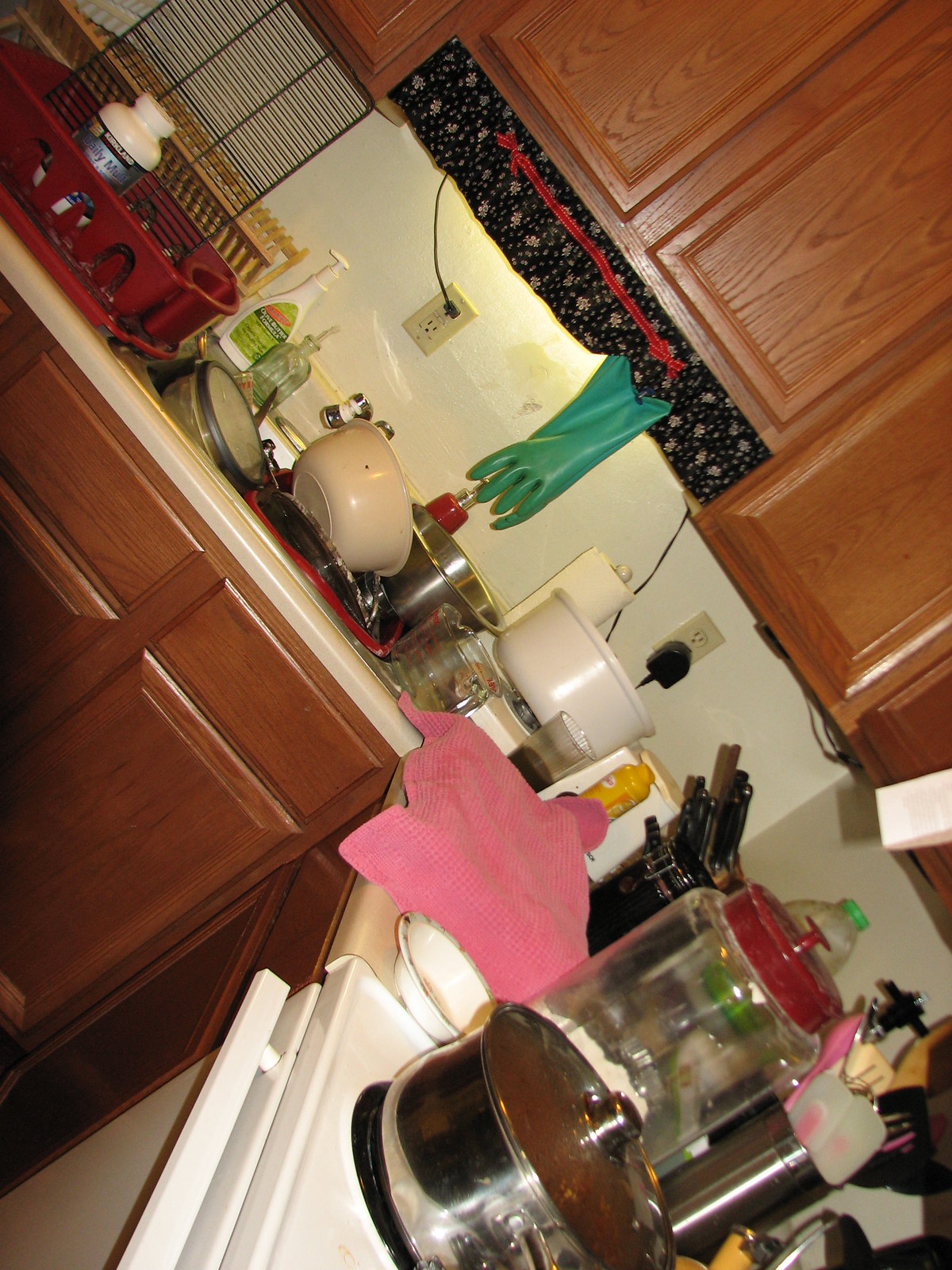This image presents a cluttered kitchen viewed from an angled perspective, emphasizing the sense of disarray. The cabinets, crafted from medium brown with a cheaper wood finish, display a grainy pattern typical of 1990s style, lacking any rustic or farmhouse charm. The plain white background serves as a minimalistic backdrop, interrupted by a few beige electrical outlets, each with appliances plugged in.

A small black valance adorned with floral designs hangs over the window. From this valance, a green dish glove with its fingers outward dangles, presumably for quick access when handling hot water, accented by a small red ribbon on top.

The kitchen sink is laden with an assortment of dirty dishes, with a red drying rack sitting nearby, cluttered with items including what appears to be a pill bottle. Bowls and cups, some still partially filled with liquids, crowd the area.

A pink towel, partially draped over an unidentified object on the counter, adds to the chaotic atmosphere. Beside it rests a small plastic bowl, and in the background, a white stove features a pot with a lid. Additionally, a drawer is slightly ajar, and a container holds various wooden spoons, spatulas, and stirring utensils, further contributing to the overall mess. The countertops are densely packed, emphasizing the lack of organization in this kitchen.